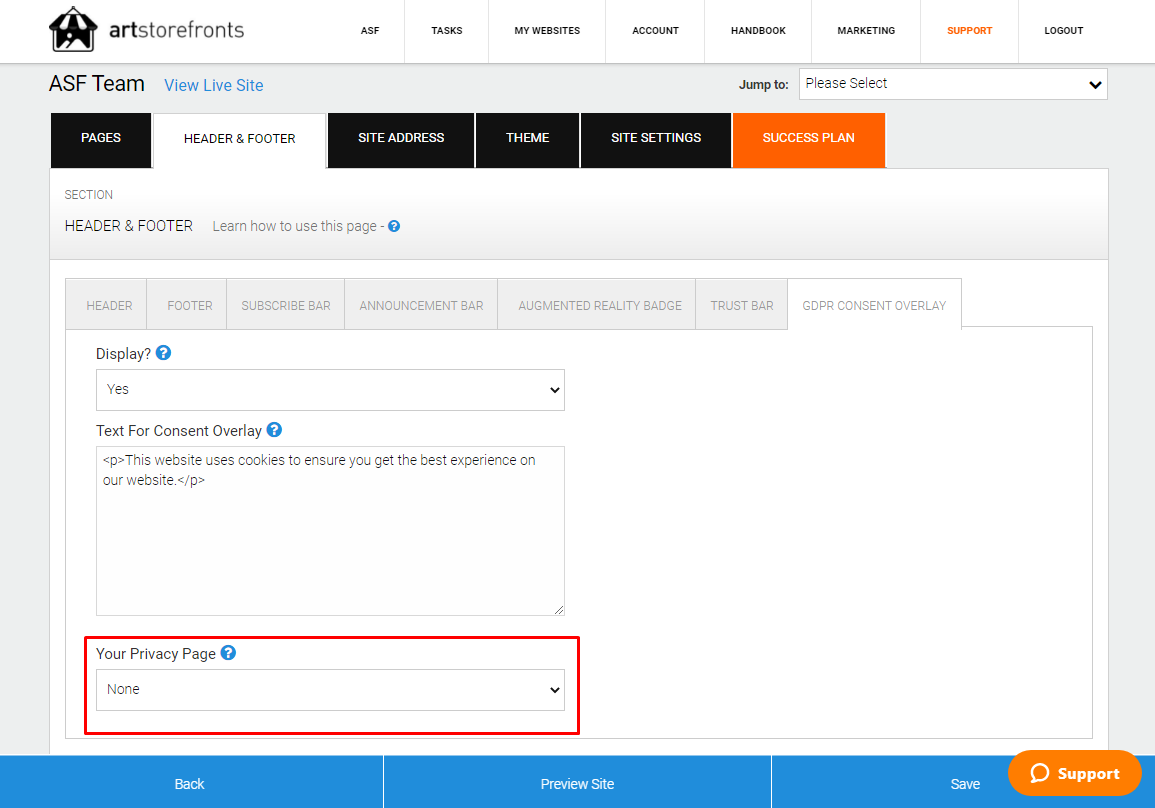This image depicts a detailed screenshot of the settings page for an Art Storefronts website. The interface features a clean design with a primary color scheme of orange and blue, complemented by white and light gray backgrounds.

At the top of the page, a white menu bar houses several navigation options: ASF Tasks, My Website, Account, Handbook, Marketing, Support, and Log Out. Directly beneath this menu, the page header reads "ASF Team" and includes a link to "View Live Site." Nearby, a dropdown menu labeled "Jump To" is set to "Please Select."

The main content area is organized into various sections and tables. A series of links at the top of a table offers navigation to different settings: Pages, Header & Footer, Site Address, Theme, Site Settings, and Success Plan. A section titled "Header & Footer" includes text that prompts users to "Learn how to use this page."

Further down, additional tabs are available within another table: Page Header, Footer, Subscribe Bar, Announcement Bar, Augmented Reality Badge, Trust Bar, and GDPR Consent Overlay. Within the GDPR Consent Overlay settings, there is an option labeled "Display: Yes" and a text box that outlines a cookie consent message: "This website uses cookies to ensure that you get the best experience on our website," formatted in a coding style. A red-outlined section states "Your Privacy Page" and is currently set to "none."

The bottom of the page hosts three blue buttons with white text: Back, Preview Site, and Save. A "Contact Support" button is also available at the bottom right corner of the interface.